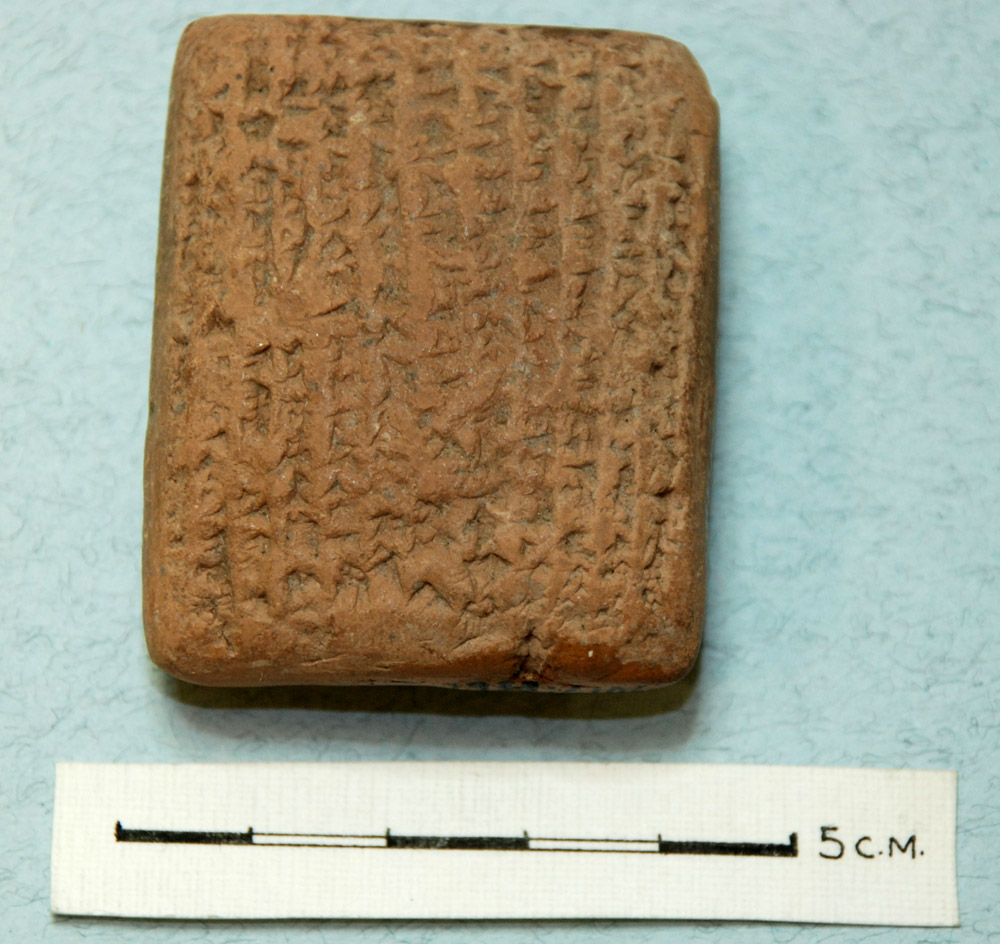The image displays a light brown, rectangular object with rounded edges, resembling a brownie, brick, or cookie, positioned on a light green surface. This surface features what appear to be hair-like details. The object itself is characterized by numerous small engravings or markings that give it a textured appearance, reminiscent of ancient text or encryptions. Below the object, there is a measuring device resembling a piece of white paper with alternating black and white bars, alongside a notation indicating "5 cm," suggesting the object’s dimensions are about 4 centimeters wide and 5 centimeters tall. The close-up view emphasizes the texture and detailed impressions on the object’s surface.